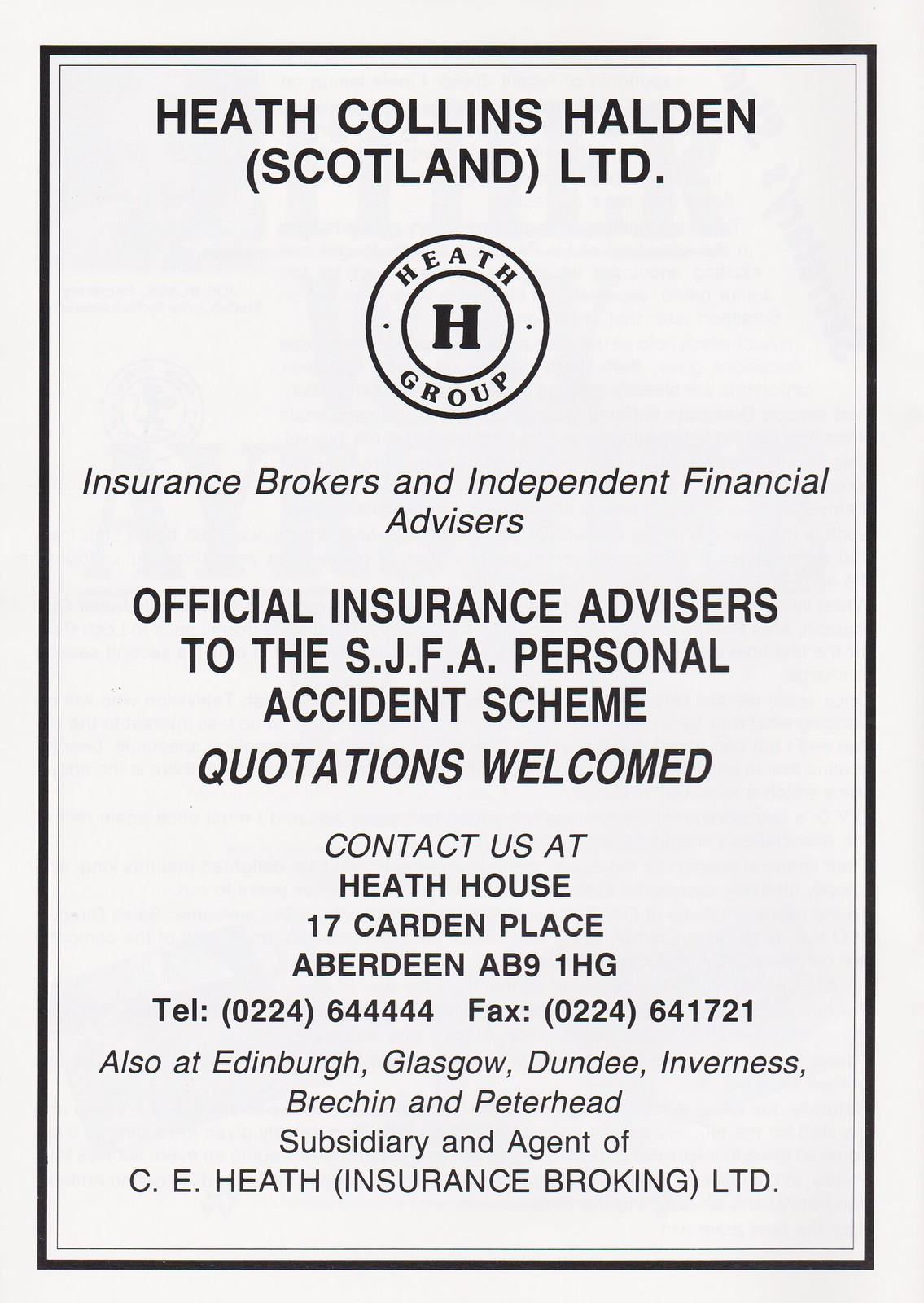The image is a scan of a pamphlet for an insurance broker seminar. It features a clean, white background with detailed, black text. At the top, it prominently displays "Heath Collins Halden, Scotland Limited" followed by the Heath Group emblem – a circular design with the letter 'H' in the center and "Heath Group" inscribed above and below it. The pamphlet identifies the company as "Insurance Brokers and Independent Financial Advisors."

Centrally positioned in bold, larger black text are the words "Official Insurance Advisors to the SJFA Personal Accident Scheme, quotations welcome." Beneath this, the contact information is detailed, listing the address as Heath House, 17 Cardon Place, Aberdeen AB9 1HG, accompanied by multiple telephone and fax numbers. The pamphlet also includes a list of other locations where the company operates such as Edinburgh, Glasgow, Dundee, Inverness, Gresham, and Peterhead. At the very bottom, in slightly smaller print, it notes that the company is a "subsidiary and agent of CE Health, Insurance Broking Limited."

The design is bordered by a thin black line, accentuating the organized layout of the information.